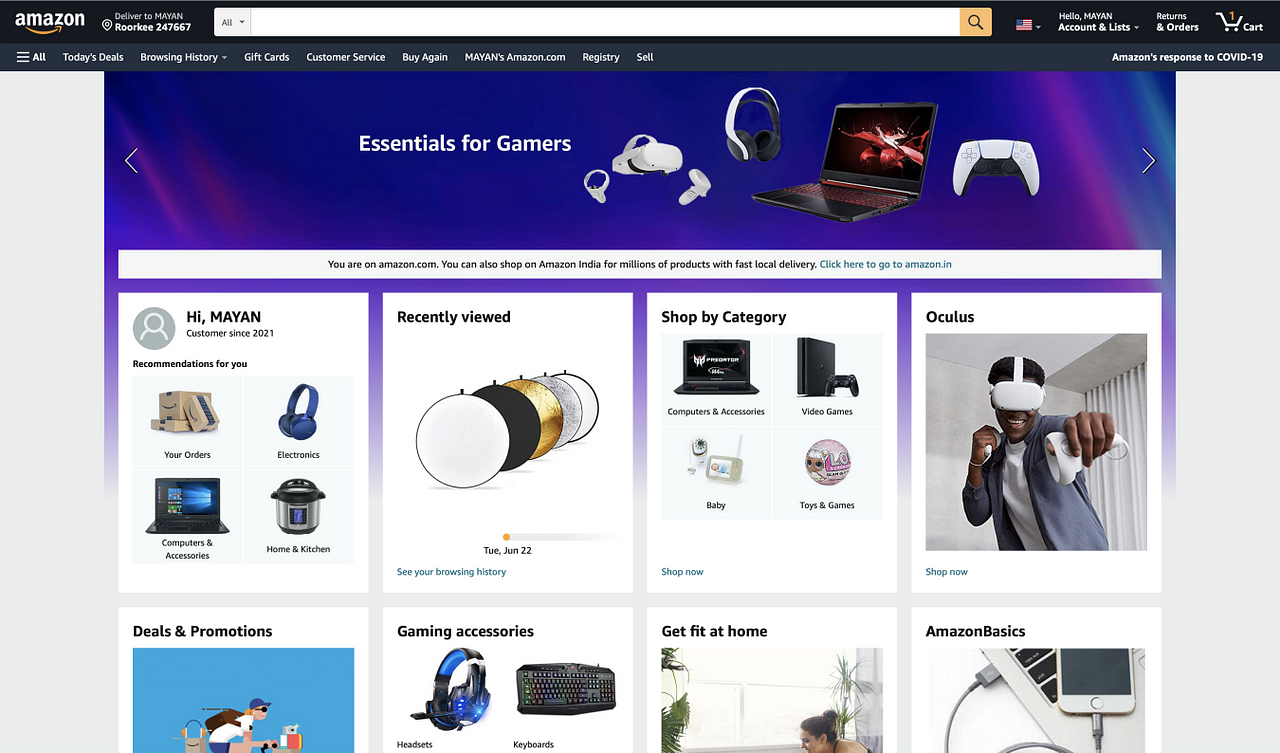This is a detailed screenshot of the Amazon.com homepage. At the very top, there are two horizontal bars: a black one and a dark gray one. The black bar at the top features the Amazon logo on the left, followed by the delivery location which is too small to read. The search field right next to it is currently blank. To the right of the search bar is an American flag icon, followed by the greeting "Hello, [Name], Accounts & Lists," "Orders," and an icon indicating one item in the cart.

Below these bars, there's a horizontal menu listing "Today's Deals," "Browsing History," "Gift Cards," "Customer Service," "Buy Again," "[Name]'s Amazon.com," "Registry," and "Sell." On the far right, there's a notice about "Amazon’s response to COVID-19."

The main header section includes a wavy graphic with a color smear, promoting essentials for gamers. Featured prominently are white Quest 2 VR headsets, a black gaming laptop, and what appears to be a Sony PlayStation 5 controller.

Below this, four horizontal columns are visible. The first column says "Hi Mayan, Recommended for You" with suggested products. The second column displays "Your Orders," the third highlights "Today's Budget Boxes" featuring items like headphones, a laptop, and what might be a rice cooker, though the image is unclear.

A further section shows "Recently Viewed" items, which include reflective panels in white, black, silver, and gold color variations. The section "Shop by Category" features various categories, such as laptops and gaming options. Oculus has its dedicated panel followed by additional four panels: "Deals and Promos," "Gaming Accessories," "Get Fit at Home," and "Amazon Basics."

Overall, the screenshot captures a comprehensive overview of the Amazon homepage layout, highlighting top navigation bars, promoted products, and user-specific recommendations.